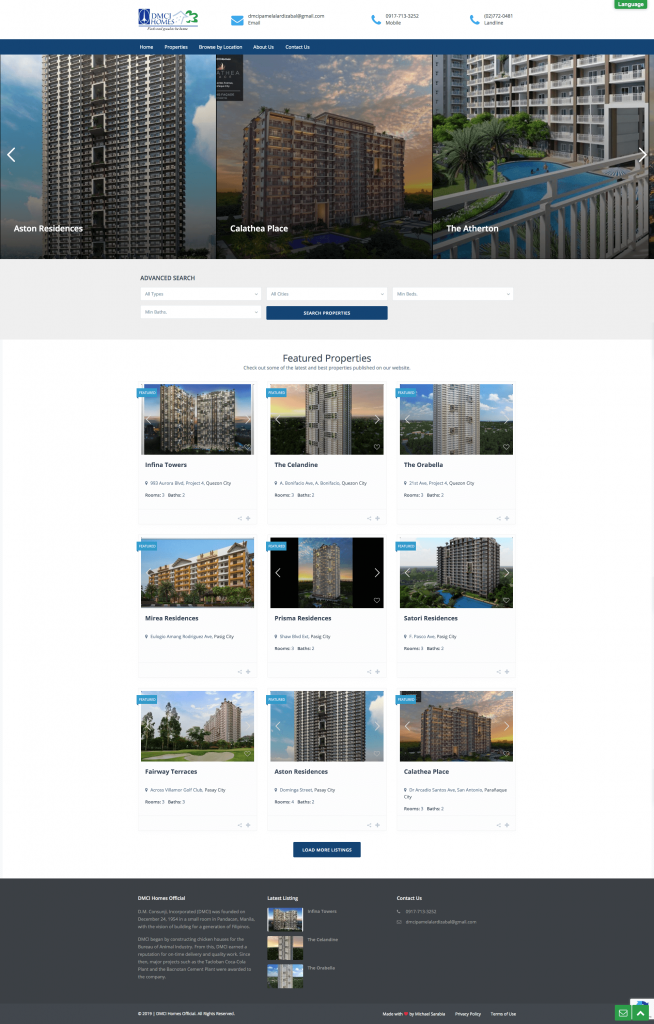The promotional website features several high-rise and upscale urban apartment buildings available for rent, specifically targeting those in downtown areas. Prominently displayed at the top of the page are three highlighted properties: Aston Residence, Calathea Place, and The Atherton, each represented by an individual image from left to right. Below these top listings, the page showcases an additional six featured properties, although the names of these buildings are not easily readable due to small text. The website includes several interactive elements, such as blue buttons with white text that serve as call-to-action prompts. Additionally, a green rectangular button located at the top left corner of the page—presumably for language selection—features white lettering. This thoughtfully designed interface aims to attract potential renters by highlighting key properties and providing intuitive navigation options.